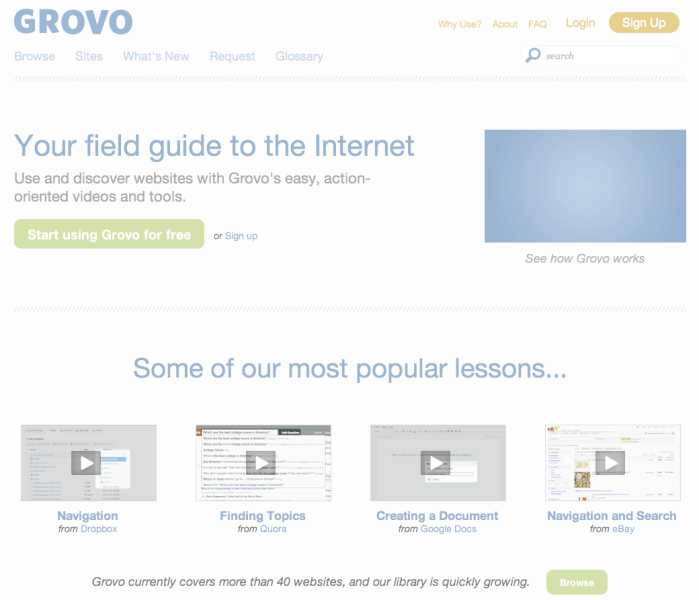**Screenshot of the GROVO Web Page**

This screenshot showcases the GROVO webpage, with the name "GROVO" prominently displayed in bold blue font across the top. The entire page appears to have a slight overlay, making the text slightly harder to read.

In the upper right corner, there are five clickable categories: About, FAQ, Login, and Sign Up. Below these options, a search bar is conveniently positioned.

Directly beneath the "GROVO" heading, there is a series of navigation links: Browse, Sites, What's New, Request, and Glossary. Below these links, a bold horizontal bar separates the top navigation from the main content.

The central feature on the page is a large tagline: "Your Field Guide to the Internet." Underneath, a subheading reads, "Use and discover websites with GROVO's easy action-oriented videos and tools."

A prominent green bar below urges users to "Start Using GROVO for Free," with a smaller blue text option nearby to "Sign Up." To the right of this call-to-action is a blue rectangular box with text inviting viewers to "See How GROVO Works," although the box lacks an accompanying image.

In the bottom half of the page, there is a section titled "Some of Our Most Popular Lessons." This section features four boxes, each containing a video player icon and a clickable rectangle. The lessons included are:
1. "Navigation from Dropbox"
2. "Finding Topics from Quora"
3. "Creating a Document from Google Docs"
4. "Navigation and Search from eBay"

Beneath these lesson boxes, there is a note stating, "GROVO currently covers more than 40 websites and our library is growing quickly," followed by a green button prompting users to "Browse."